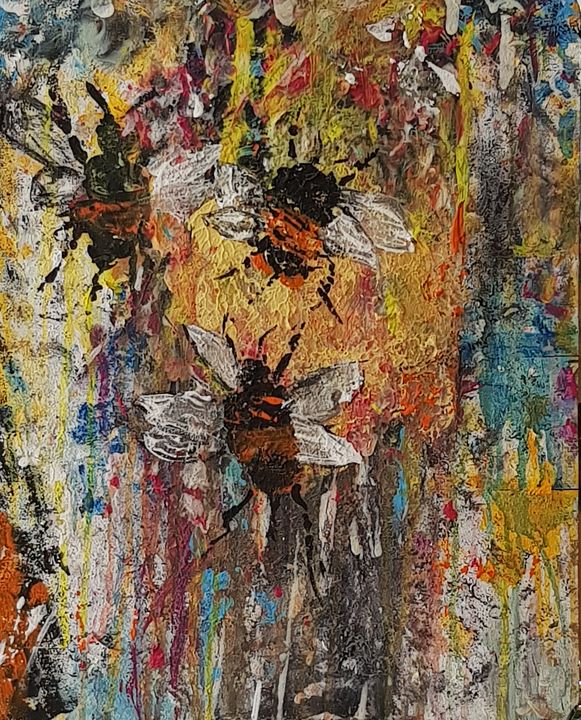This abstract painting features a dynamic and vivid background composed of a variety of colors, including yellow, red, blue, white, green, purple, orange, black, gray, and teal, all smudged together in layered stripes and splotches to create an energetic, almost chaotic canvas. Prominently displayed within this colorful backdrop are three bee-like insects with distinctive black heads and bodies bearing orange stripes. Each insect has six black legs - two pointing upwards and four downwards - and two pairs of white, faintly outlined wings. The placement of the insects is notable: one is positioned at the top left of the frame, another at the center top, and the last one at the center middle bottom. While the top central insect faces the viewer, the bottom one is shown from the back in a flying position. The top left insect also faces the viewer, contributing to a balanced and intriguing composition. Additionally, near the bottom right corner, about an inch from the edge, there is a small, yellow star-like shape that adds an extra element of interest to the artwork.